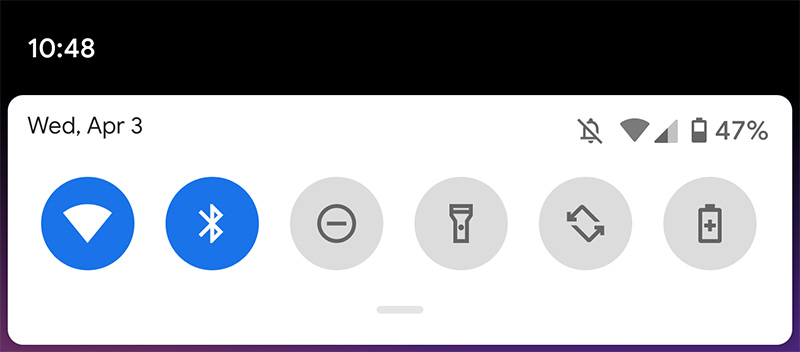The image is a screenshot capturing a segment of a screen, primarily focusing on the top header or banner. The background is a solid black, contrasting with a small, white pop-up box located in the upper left corner. The digital time displayed in white text reads "10:48." Directly below the time, within the white pop-up, is the date "Wednesday, April 3rd" written in dark gray text. 

To the right of this pop-up box, a series of status icons are lined up. First, there's a notification icon indicating that notifications are off. Next is the Wi-Fi icon, signifying that Wi-Fi is currently on. Following that is a battery icon, which shows the battery level at 47%.

Below this top section, there are large circular icons arranged horizontally, intended for quick access to various functions. The first is a blue circle featuring a white Wi-Fi icon. Adjacent to it is another blue circle displaying the Bluetooth icon. Moving further to the right, there is a gray circle with a flashlight icon, and lastly, a gray circle containing a battery icon.